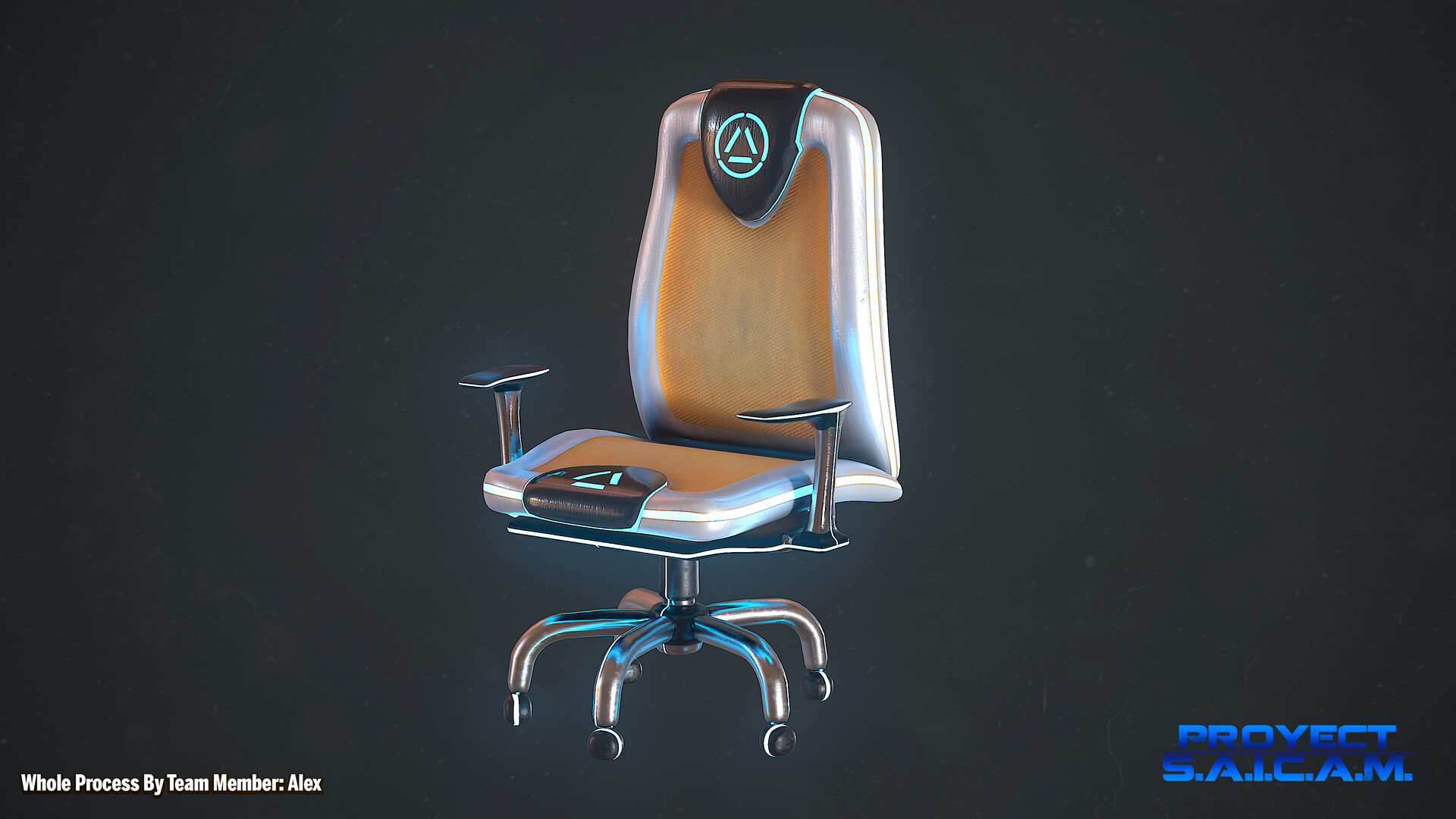The image showcases a modern, high-tech gaming chair with an office-style design. The chair sits on a sturdy metal base with five wheeled legs, somewhat resembling octopus legs. Its seating area and backrest feature a brown mesh material bordered by gray accents. Prominently, there are two glowing blue triangles on black fabric—one on the seat and another on the headrest. These illuminated symbols add a futuristic touch. The chair also has silver metal armrests with black padding for comfort. The background of the image is a solid dark gray, giving emphasis to the chair. Text in the lower left corner reads "Whole process by team member Alex," while the lower right corner displays the project name "S.A.I.C.A.M." in a blue, watermark style.